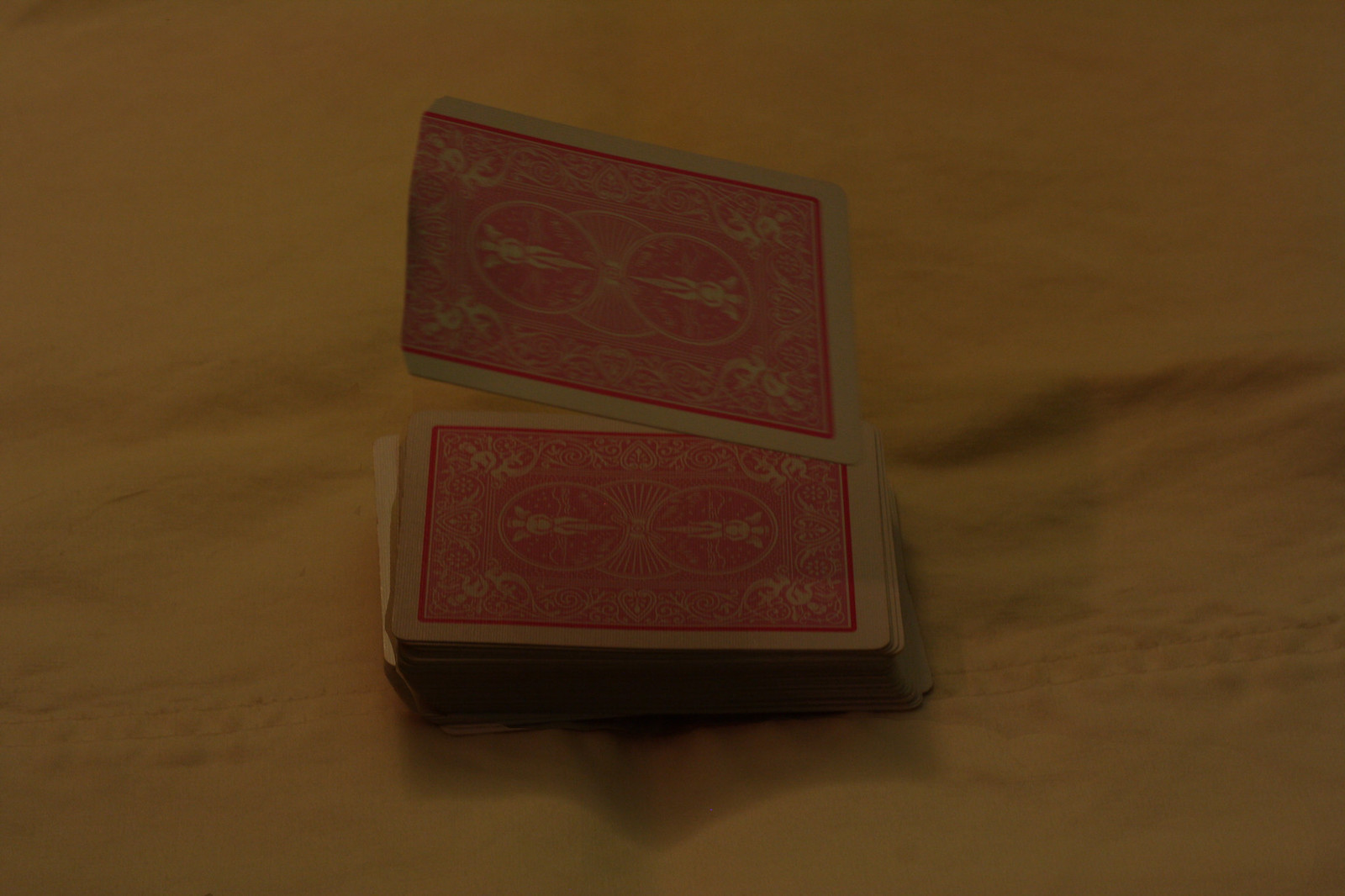This photograph captures a detailed scene featuring a deck of Bicycle brand playing cards resting on a rumpled, golden-colored cloth. The iconic red and white pattern with a vintage bicycle logo, characteristic of this well-known brand, is clearly visible on the deck. Interestingly, one card appears to be either mid-fall onto the deck or possibly levitating just above it, hovering at a slight angle rather than perfectly horizontal. This card stands out not only for its positioning but also because its upper edge lacks the usual white border. Instead, it appears to have been cut and possibly singed, as indicated by a brown stain along the top edge. The contrast between the pristine design of the deck and the altered, floating card adds an intriguing element to the composition.